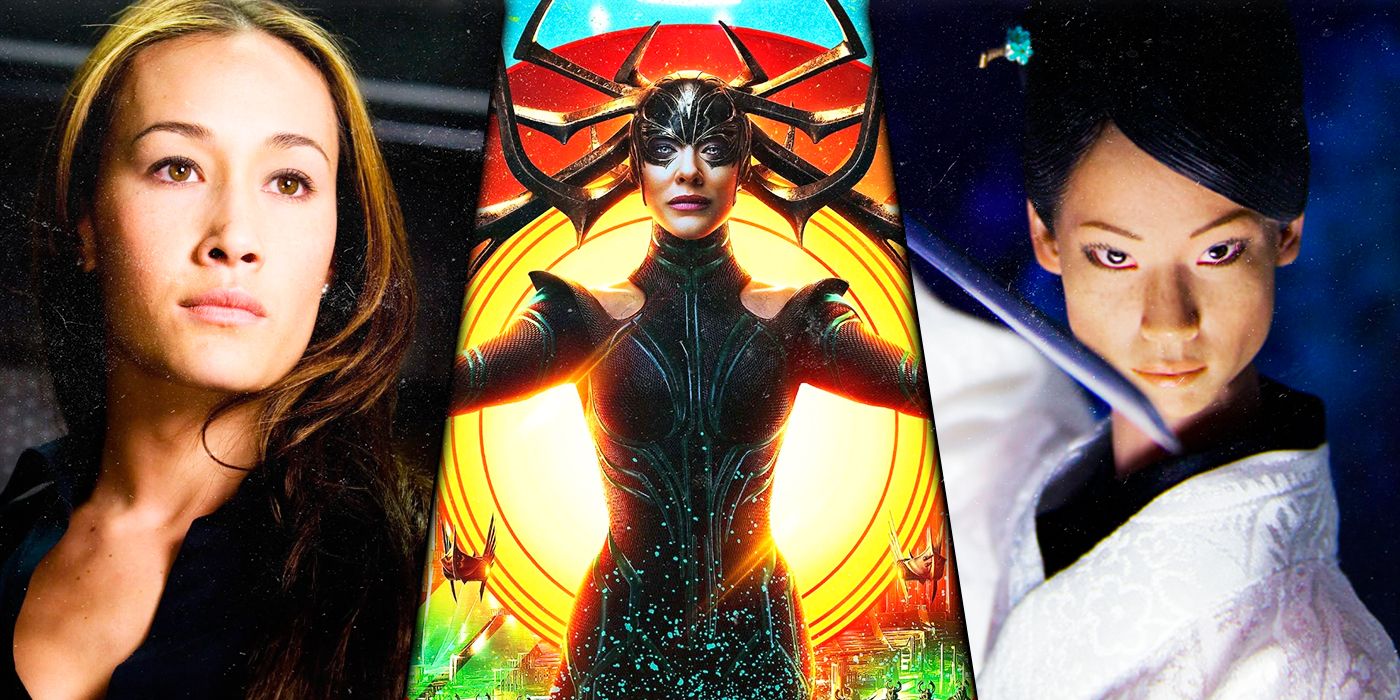This detailed image resembles a movie poster featuring three distinct female characters, possibly from the same film. The leftmost character is a woman with dark hair accentuated by blonde highlights and brown eyes, dressed in a low-cut black shirt. She gazes thoughtfully into the distance. The central figure, a recognizable yet unplaceable character, is dressed in a tight, black, shoulder-baring outfit adorned with pronounced black epaulets. She wears a black headdress that covers her eyes, extending into antler-like protrusions, set against a backdrop of red and yellow circles with green at the bottom. On the right is another woman with almond-shaped, blue eyes. Her dark hair is parted and pulled back behind her ear, revealing a serious, menacing expression. She holds a Japanese sword and is clad in a white karate gi overlaying a black shirt. The image blends elements of sci-fi and martial arts, suggesting a unified theme across the characters.